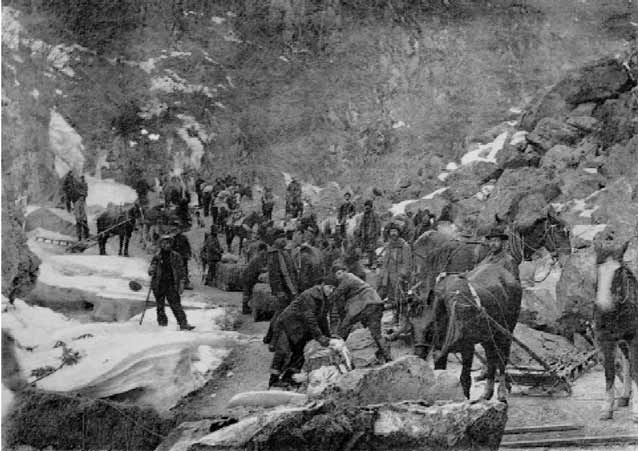"A sepia-toned photograph from the late 19th to early 20th century captures a rugged mountain expedition. The image, grainy and slightly pixelated, portrays a group of workers, possibly gold prospectors or stone miners, laboring up a rocky mountain trail. Men outfitted in long coats, long pants, and hats, typical of the era, wield pickaxes and other digging tools. Horses draped with gear and harnesses accompany them, each carrying essential supplies. The jagged, rocky terrain and the distant mountain outline suggest an arduous journey. The scene, steeped in the essence of hard labor, is a testament to the relentless spirit of the pioneering era."